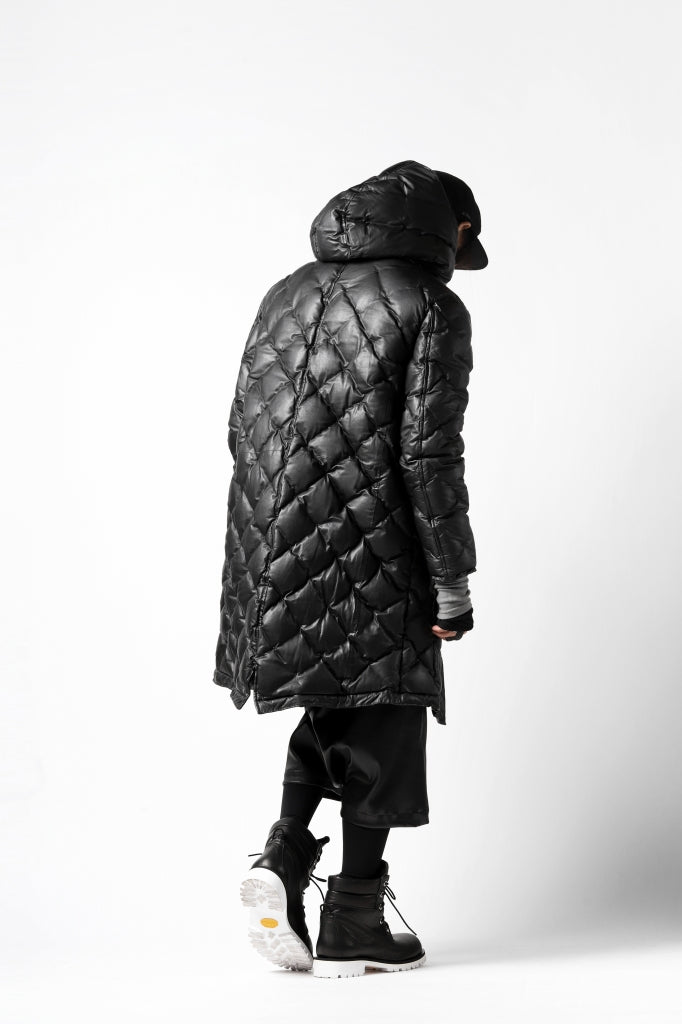The image is a black-and-white photograph with selective color that depicts the backside of a male figure walking towards the right side of the frame, with his head bowed. The composition captures him from the top of his head to the bottom of his shoes. The background is a light gray gradient with subtle white tones, and the photo is presented in a vertical rectangular format. He is dressed in a black, knee-length quilted coat with a hood that is not up, giving the coat a diamond-shaped textured pattern.

He wears a black baseball cap, visible by the side of the brim, and beneath the coat, a gray sweater can be glimpsed. The coat has a central slit at the hem, revealing a bit of his attire underneath, which includes long, flared black shorts and either black tights or trousers. His shoes are black with distinct white soles, notable for an orange circle in the middle of the sole on the raised boot. 

His right hand extends from his sleeve, slightly curled as if forming a fist, and is colorized at the fingertips in the otherwise monochromatic image. Additionally, white wrappings are seen around his wrists. This highly detailed and realistic photograph captures the subject in an almost representational artistic style, where each element from the texture of the coat to the precise color details on his hand and shoes is meticulously depicted.